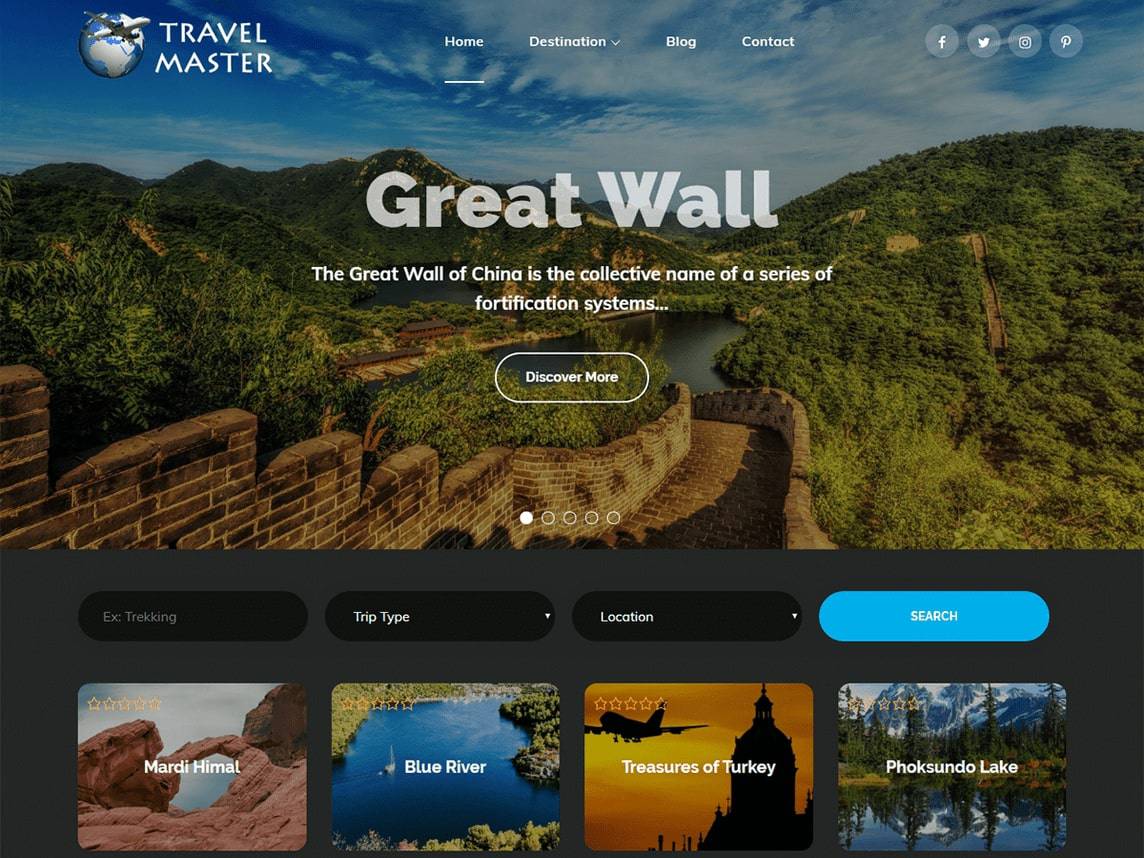The advertisement from Travel Master features a prominent logo in the upper left corner, showcasing a globe with a jet plane circling it. To the right of this logo, written in a slender, white, capitalized font, is the name "Travel Master." Just below are navigation buttons labeled "Home," "Destination," "Blog," and "Contact," with corresponding social media icons for Facebook, Twitter, Pinterest, and an additional unidentified icon.

Covering the top section of the ad is a panoramic image of the Great Wall of China, highlighted against a backdrop of blue skies, rolling green hills, and white clouds. In bold white letters at the center, the title "Great Wall" is displayed, with the accompanying text, "The Great Wall of China is the collective name of a series of fortification systems..." Beneath this text, a rectangular button encourages viewers to "Discover More."

Further down, the ad features a sleek navigation bar with categories "Trekking," "Trip Type," "Location," and a pale blue "Search" button. Below this, four smaller clickable images represent various destinations offered by Travel Master: 

1. **Mardi Himal:** Depicts a distinctive pinkish rock formation set against a blue and white sky.
2. **Blue River:** Shows a stunning blue waterway surrounded by lush greenery, with a small isthmus extending off to the right.
3. **Treasures of Turkey:** Captures a tall church tower silhouetted against a golden sky, with an airplane visible on the left.
4. **Fuxundo Lake:** Displays a glistening lake that mirrors the sky, mountains, and tall green trees in the background.

The detailed layout and vivid imagery vividly promote Travel Master’s array of exciting travel destinations.